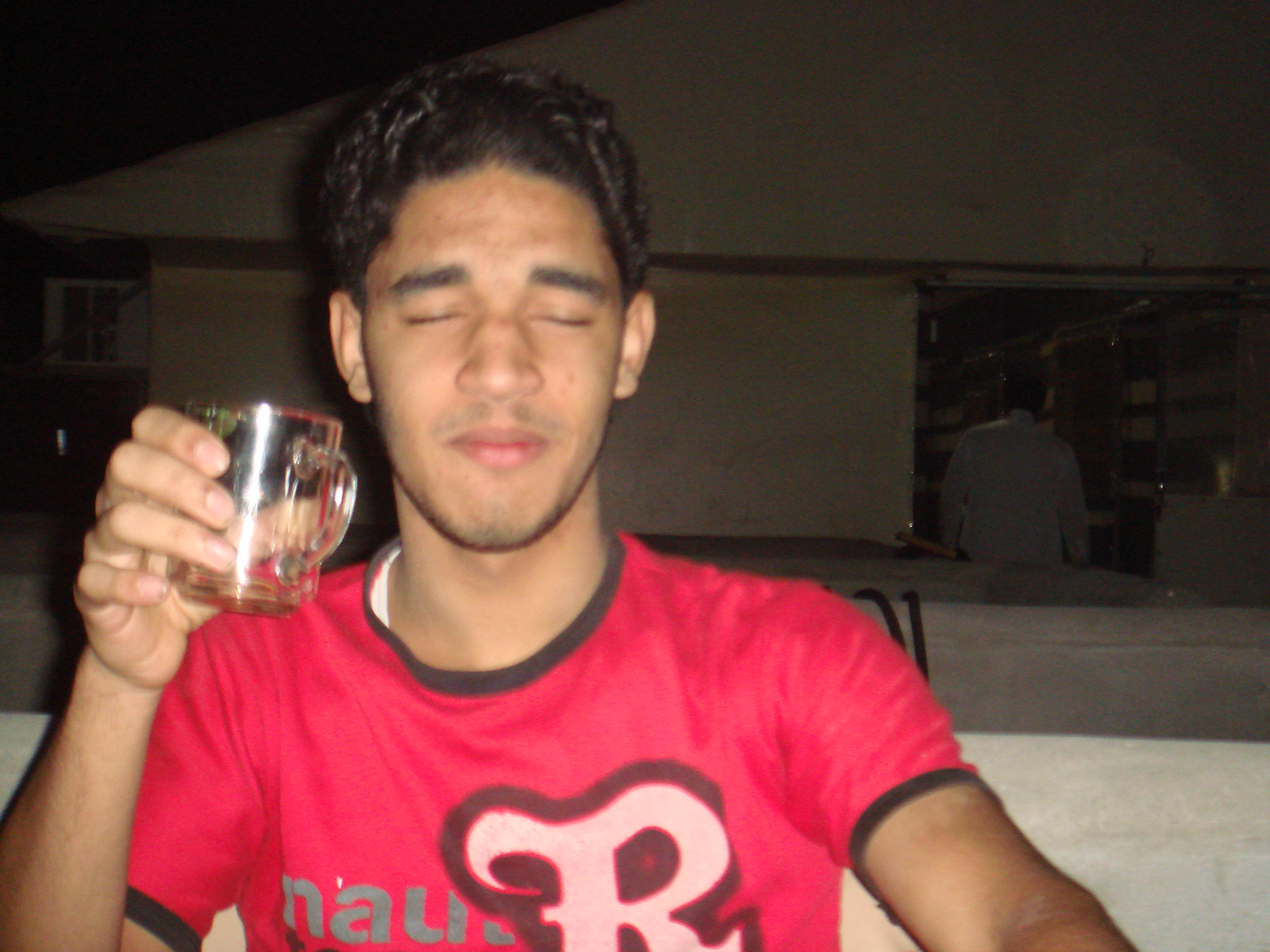The photograph depicts a young man, possibly in his 20s, with caramel-colored skin and short black hair styled back on his forehead. He is wearing a red t-shirt with black and gray trim around the collar and sleeves, prominently featuring a large white letter "R" on it. His eyes are closed, and his lips are pursed, suggesting he may have just taken a drink from the clear, empty glass with a handle he is holding in his right hand, positioned to the left of the image.

In the background, the upper half shows the side of a tan house, with an air conditioning unit visible on the left. There is also an open door where another person, wearing a white long-sleeve shirt, can be seen with their back facing the camera. The setting appears to be nighttime, suggesting a relaxed, casual gathering, possibly a selfie taken near a friend's house.